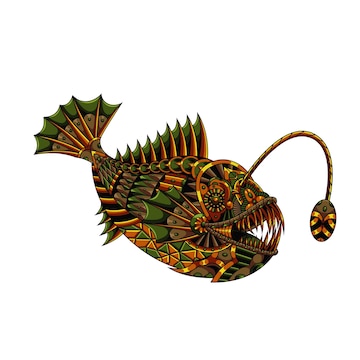This image depicts a detailed, vector art piece of a lanternfish, composed of small, colored pieces reminiscent of a mosaic. The fish is shown in a side view, facing to the right against a plain white background. The overall color scheme includes intricate patterns of green, orange, yellow, black, and brown distributed across its body. The lanternfish's mouth is slightly open, revealing long, sharp teeth. Prominently featured is a long filament emitting from the center of its head, ending in an oval object with yellow, black, and brown hues. The fish's fins and tail are characterized by gold spines with green and black membranes in between. Noteworthy are its small, inlaid eyes, featuring green and orange stones arranged in a circle. The fish’s structure and vibrant color patterns evoke a sense of artistic complexity, making it resemble a piece of decorative art.